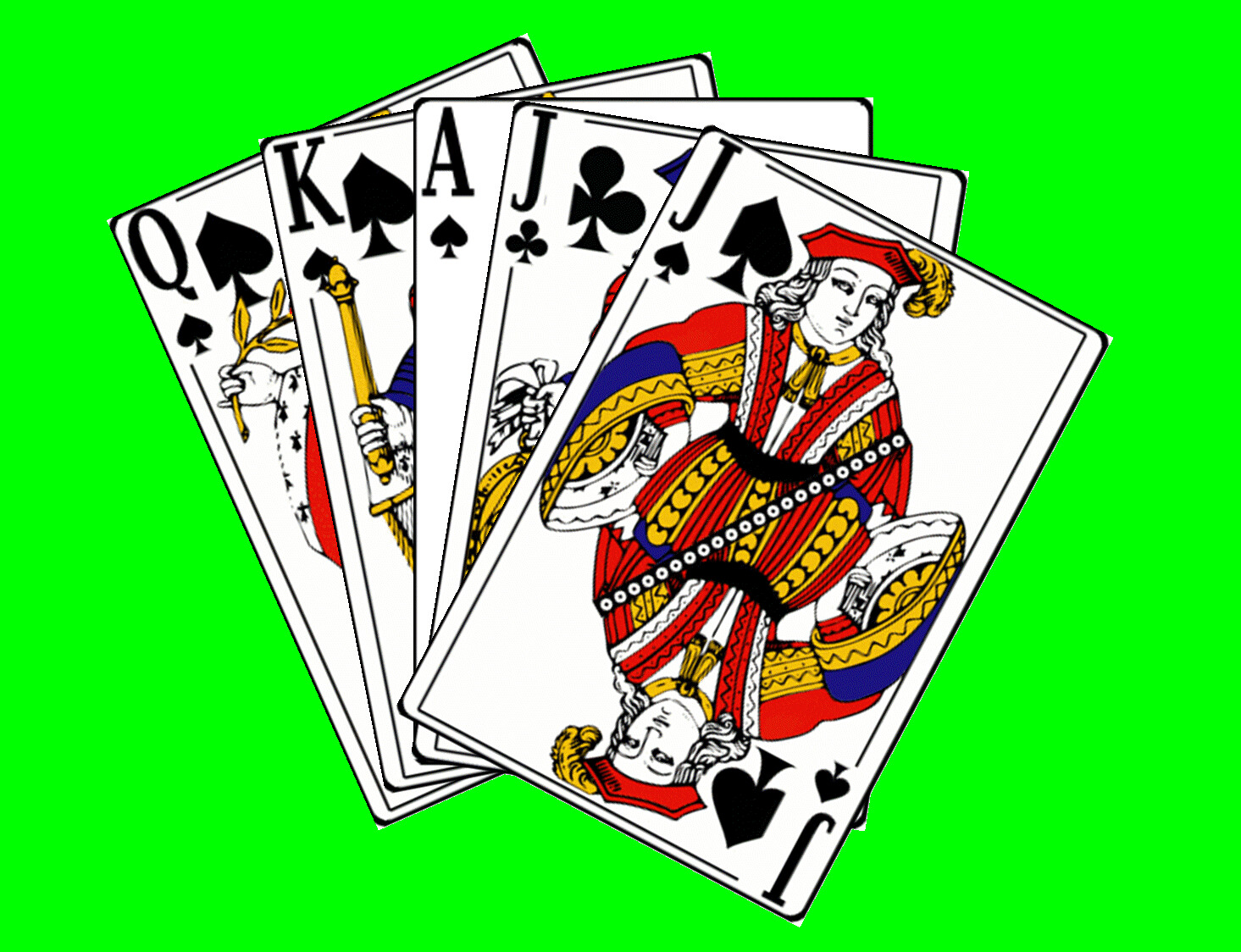The image features a set of five prominently large playing cards arranged against a very light green background. Each card displays intricate artwork and vibrant colors. 

1. **Queen of Spades (Q)**: This card showcases a detailed depiction of a queen. She dons a red coat with white outer linings, complemented by white gloves. In her hand, she holds a gold branch. The card includes the spade icon in both a small and a larger form.

2. **King of Spades (K)**: The king is illustrated in a royal blue coat while holding a gold stick. The card also displays two spade icons and a bit of an additional element resembling a yellow stick held by someone in part of the depiction.

3. **Ace of Spades (A)**: The ace is presented centrally with its iconic single spade symbol, simple yet bold in black, dominating the card.

4. **Jack of Clubs (J)**: This card highlights a jack of clubs, symbolized by the three-leaf clover design. The jack is adorned in a coat of red, blue, and gold, sporting a remarkable hat with a red base and a yellow feather. The face is rendered in black and white with visible hair, and the imagery features a reflective, mirroring effect on the card.

5. **Jack of Spades (J)**: Similar to the previous jack, this card shows a jack adorned similarly in a red, blue, and gold coat, with a distinguishing red hat and yellow feather. 

Each card is depicted with a high level of detail, making the figures and symbols particularly striking against the subtle green backdrop.